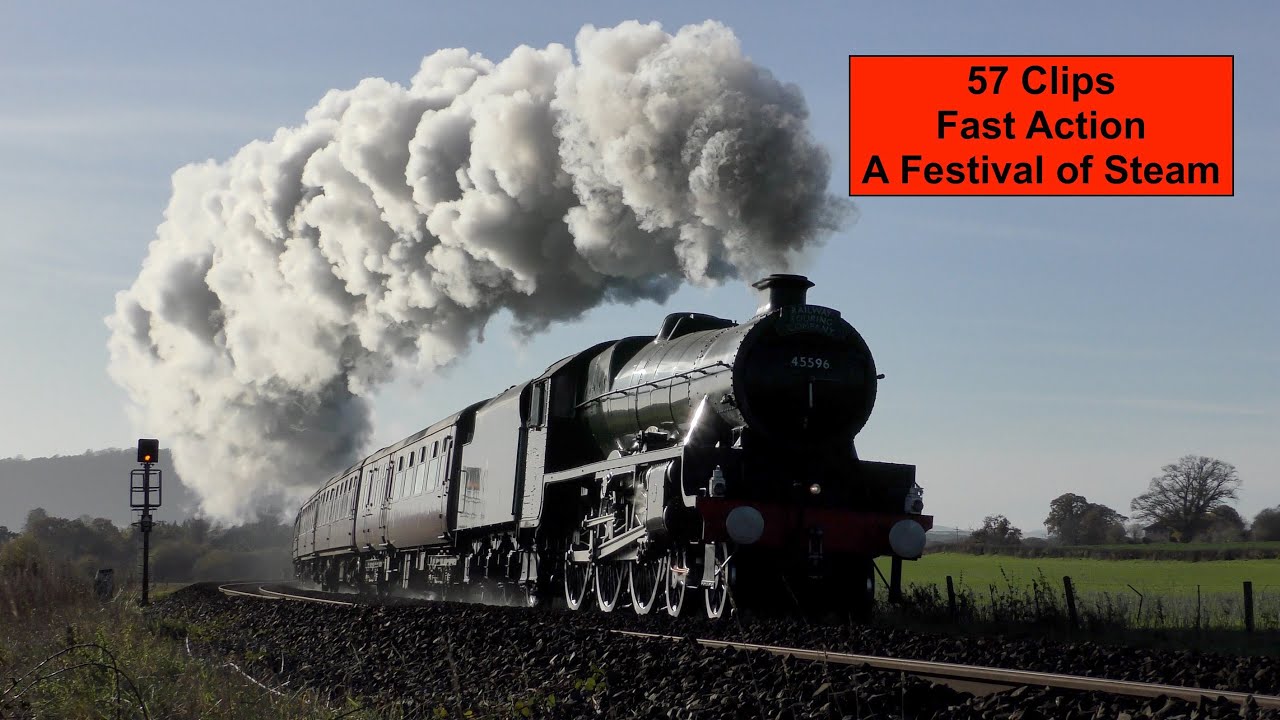The image is a digital photograph of a black steam train with the number 45596, puffing large plumes of gray and white smoke from its smokestack as it travels from left to right down a gravelly railway track. The scene is set on a sunny day with clear blue skies and scattered light clouds. The landscape features wide open green fields and dark green trees in the background, with a distant hill range on the left side and some bare trees along the horizon. A train signal with a yellow light is visible near the tracks, signaling the passage of the train. The inset in the top right corner of the image displays a red rectangular box with black text that reads "57 Clips, Fast Action, a Festival of Steam," suggesting the picture might be a promotional thumbnail or advertisement. The overall light captures most of the train, casting shadows on the ground while illuminating the train's features distinctly against the bright, natural backdrop.